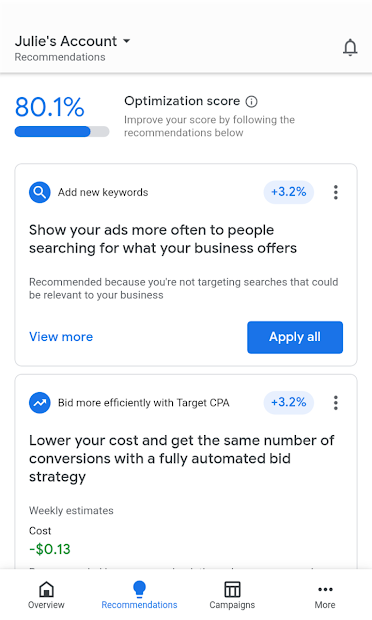The mobile screenshot displays a screen from an app called Julie's Account. At the top left corner, the name "Julie's Account" is visible, while a bell icon is situated on the top right of the screen.

Below "Julie's Account" is a section titled "Recommendations," separated by a light horizontal border. Directly beneath this line, there is blue text showing "80.1%," accompanied by a blue progress bar. This is followed by the text "Optimization Score" and a note stating, "Improve your score by following the recommendations below."

Two recommendation boxes are displayed below this section:

1. The first box recommends adding new keywords. It includes a magnifying glass icon within a blue circle, and a "3.2%" improvement indicator on the right side of the same row. The heading reads, "Show your ads more often to people searching for what your business offers." At the bottom of this box are two buttons: "View More" on the bottom left and "Apply All" on the bottom right.

2. The second box suggests bidding more efficiently with a target CPA. It features an upward zigzag arrow icon next to a "+3.2%" improvement indicator on the right. The heading states, "Lower your costs and get the same number of conversions with a fully automated bid strategy." The box also includes a green "Weekly Estimates Cost" of "-0.13." 

At the bottom of the screen, a navigation header contains four icons: "Overview" represented by a house, "Recommendations" indicated by a blue light bulb, "Campaigns" symbolized by a building, and a "More" section denoted by three ellipses.